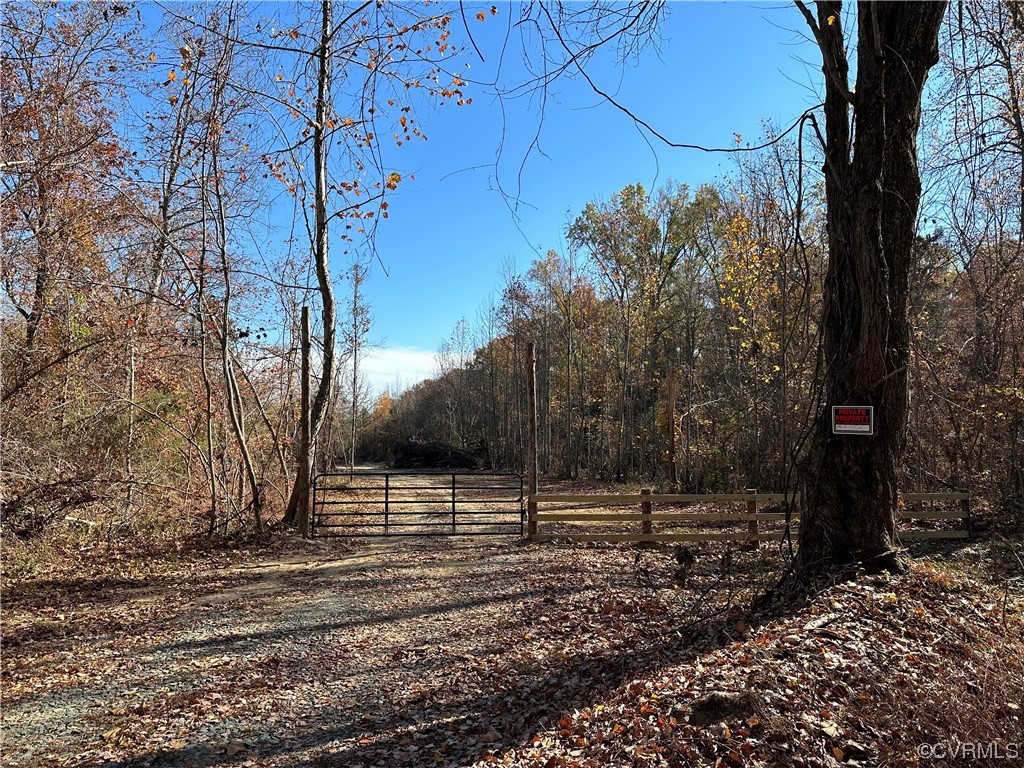This landscape color photograph, taken in the fall during the daytime, features a wide, unpaved driveway or country road composed mainly of dirt and gravel, peppered with dead, brown leaves. A striking blue sky with a light cloud cover forms the backdrop, contrasting with the foreground's earthy tones of beige, gray, and brown. The path is flanked by rows of barren trees with spindly branches, adding to the dry, desolate feel of the scenery. At the center of the image, a metal gate blocks the road, signifying private property, complemented by a large tree trunk on the right, bearing a “Keep Out” sign in red, black, and white. The ground is littered with fallen leaves, reflecting the season's transformation, while sparse green patches hint at the lingering traces of summer amidst the otherwise dry and rustic environment.